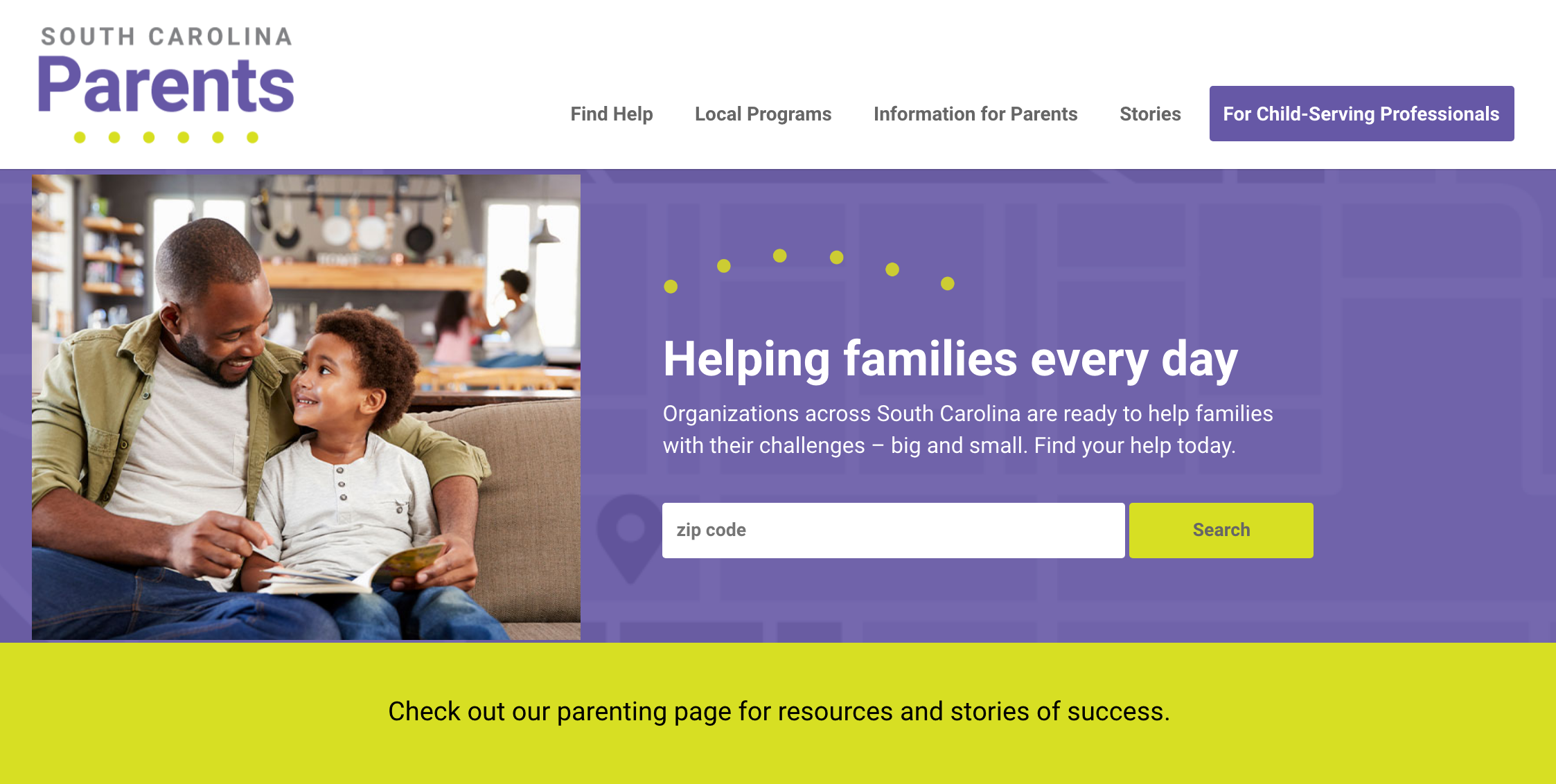A detailed descriptive caption for the image could be:

"The image is a screenshot of a website displayed on a full-width laptop or desktop monitor, showcasing 'South Carolina Parents,' a comprehensive resource for both parents and child-serving professionals. The homepage features a heartwarming photograph on the left side, depicting a father and son cuddling on a couch while reading a book. To the right of this touching image, there is informative text and a search box for users. The text reads, 'Helping families every day. Organizations across South Carolina are ready to help families with their challenges, big and small. Find your help today.' Below the text, there is a search box that prompts users to enter their zip code, against a backdrop of a grayed-out map overlaid with a light purple tint. Further down, additional text encourages visitors to 'Check out our parenting page for resources and stories of success.' The website's clean and inviting design features a color palette of white, purple, green, and accents of yellow, creating an approachable and supportive online environment for its visitors."